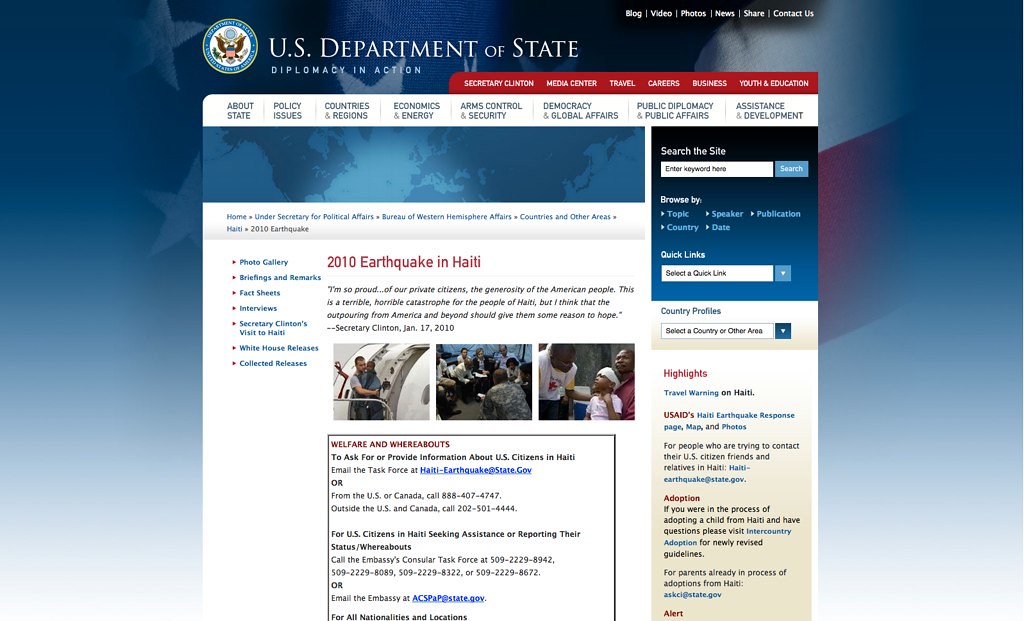This is a detailed screenshot of the U.S. Department of State's Diplomatic Inaction webpage. The interface features a prominent red tab navigation bar at the top with options labeled "Secretary Clinton," "Media Center," "Travel," "Careers," "Business," and "Youth and Education." Directly below, a white navigation bar presents additional categories: "About State," "Policy Issues," "Countries and Regions," "Economics and Energy," "Arms Control and Security," "Democracy and Global Affairs," "Diplomacy," "Public Affairs," and "Assistance Development."

Centrally displayed on the page is an image of a world map, rendered in light blue and dark blue to delineate the continents. Adjacent to the map is a search bar, followed by a headline reading "2010 Earthquake in Haiti." Below this headline are three thumbnail images showcasing ongoing relief efforts and providing links to a photo gallery and fact sheets.

On the lower section of the page, users can find a "Quick Links" area with options such as "Adoption," "USDA Alerts," and "Country Profiles," facilitating easy navigation to specific topics. The backdrop of the webpage subtly features the flag of the United States, reinforcing the official nature of the content.